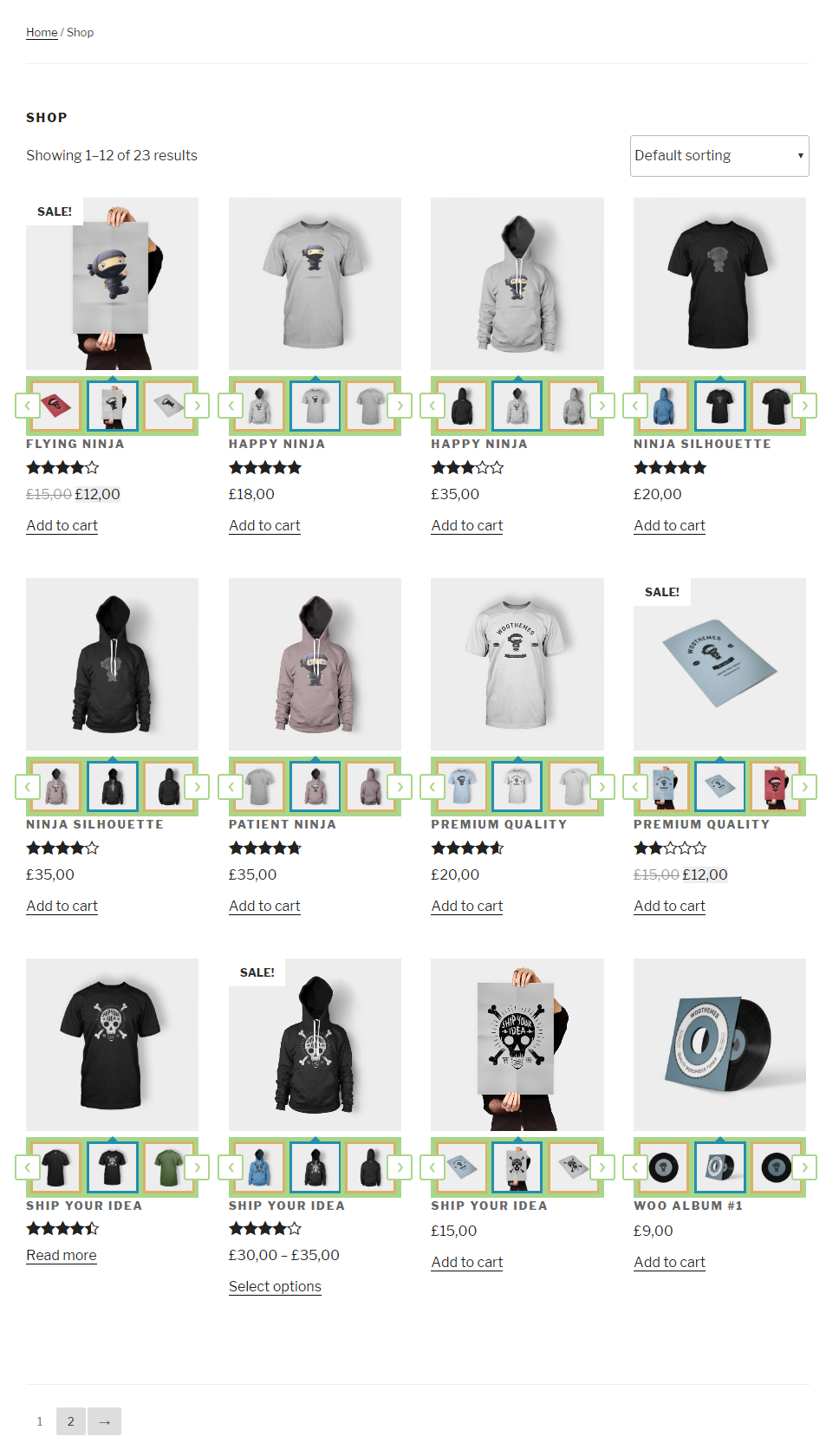This image is a screenshot of an online store's homepage. At the top, navigational options include "Home" and a heart icon labeled "Like," followed by a "Shop" section. The store indicates it is displaying items 1 through 12 out of 23 available results.

Directly below this header is a series of images showcasing various t-shirts. The first image on the left features a person dressed in black, holding a poster that obscures their face. The t-shirt beside them has the word "Sell" next to it and features a small figure wearing a bandana with most of their face covered, also dressed in dark attire.

Adjacent items include another t-shirt for sale, a hoodie, and a black t-shirt. Each clothing item displayed includes the information on available colors, offering options such as blue or other variations.

The page is formatted into three rows, each containing four items. In addition to the t-shirts and hoodies, one of the rows presents an album for purchase, described as "The Black Album" in a gray sleeve. Furthermore, a premium quality poster is also listed, notably on sale with a two-star rating.

Each product image is accompanied by a rating system, showcasing various ratings from five stars to as low as three or four stars. Overall, this online store appears to specialize in selling a combination of clothing, albums, and other miscellaneous items.